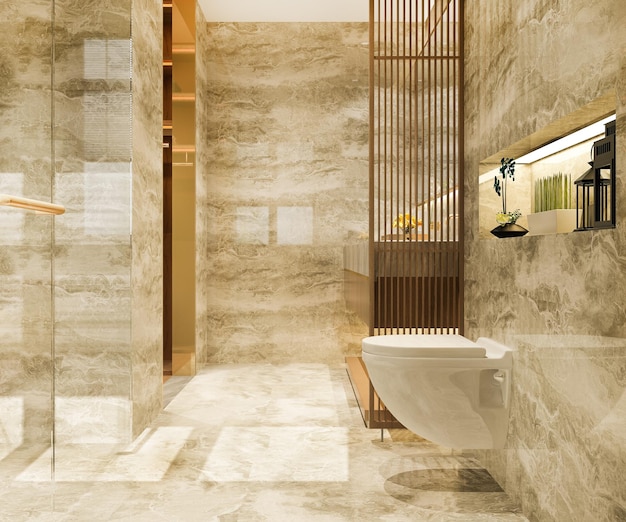This is a color photograph of a very luxurious bathroom, featuring floor-to-ceiling yellow and white marble with tints of black and goldish metallic accents. The white marble tabletop vanity area with a brown marble bottom is located at the far right corner, partially covered by a stringed wooden partition. In front of the vanity, there is a modern, wall-mounted floating white porcelain toilet. Above the toilet, there is a recessed shelf holding a white porcelain cup with plants. The roof is white, creating a bright and airy atmosphere, enhanced by natural light from an unseen window likely located in the shower area. Additional decor includes a vase with yellow flowers by the sink, and various objects like lanterns and flowers on the shelf above the toilet.